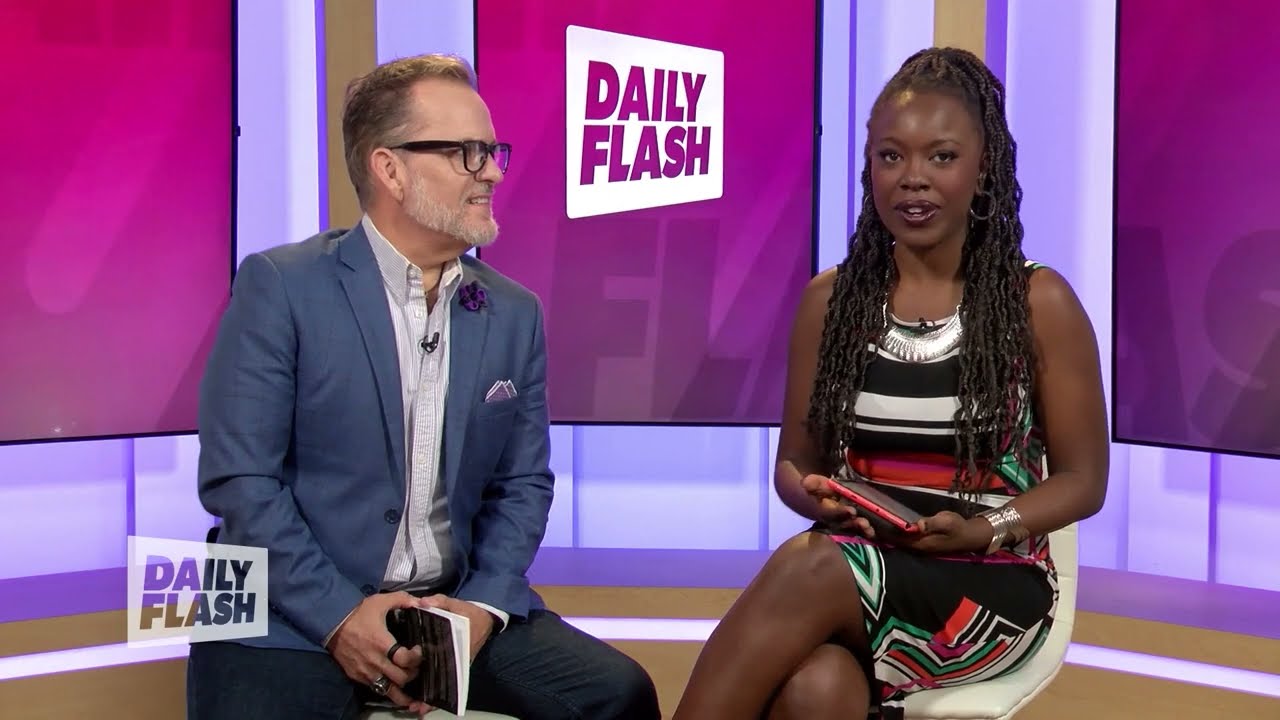The image is a still frame from a talk show called "Daily Flash," featuring two individuals seated on white stools against a purple and white backdrop. On the left, a middle-aged white man with slicked-back, graying blond hair and a light grayish beard is dressed in a dark blue blazer adorned with a purple circular pin on the lapel, an off-white collared shirt, and dark pants. He sports large black horn-rimmed glasses and holds a notebook in his crossed hands. To the right, an African-American woman with long braided hair extending past her waist is attired in a sleeveless dress with a black, white, red, and green pattern. She holds a red tablet with both hands and wears several bracelets on her right arm. Both have small microphones attached to their outfits. Behind them are vertically aligned monitors displaying the "Daily Flash" logo in dark purple text within a white square, set against a gradient backdrop transitioning from dark to light purple. The floor beneath them is brown with a white circle. The "Daily Flash" logo also appears in the lower-left corner of the image. Both hosts are engaged with the camera, seemingly in mid-conversation.